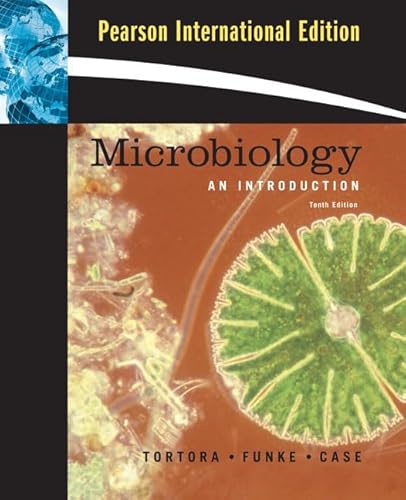The image depicts the front cover of a Pearson International Edition textbook. At the top left corner, there are two overlapping blue globe shapes. Directly to the right, a black rectangle displays the text "Pearson International Edition" in yellow font. Below this rectangle is a white arc stretching from left to right. The primary title "Microbiology" is prominently featured in black serif font centrally on the cover, followed by "An Introduction" in all capital letters beneath it. Further down, "10th Edition" is noted. At the bottom, the authors' names "Tortora, Funk, and Case" are listed in capital letters. 

The background is predominantly rusty orange with varying elements. On the left side, an image resembling a pile of white ice cubes is visible. Adjacent to it, on the right, a green circular shape, evocative of a grapefruit slice with yellow lines, is prominent. The overall appearance is detailed and visually segmented, with the top and bottom portions divided into distinct sections, each contributing to the cover's informational and decorative aspects.